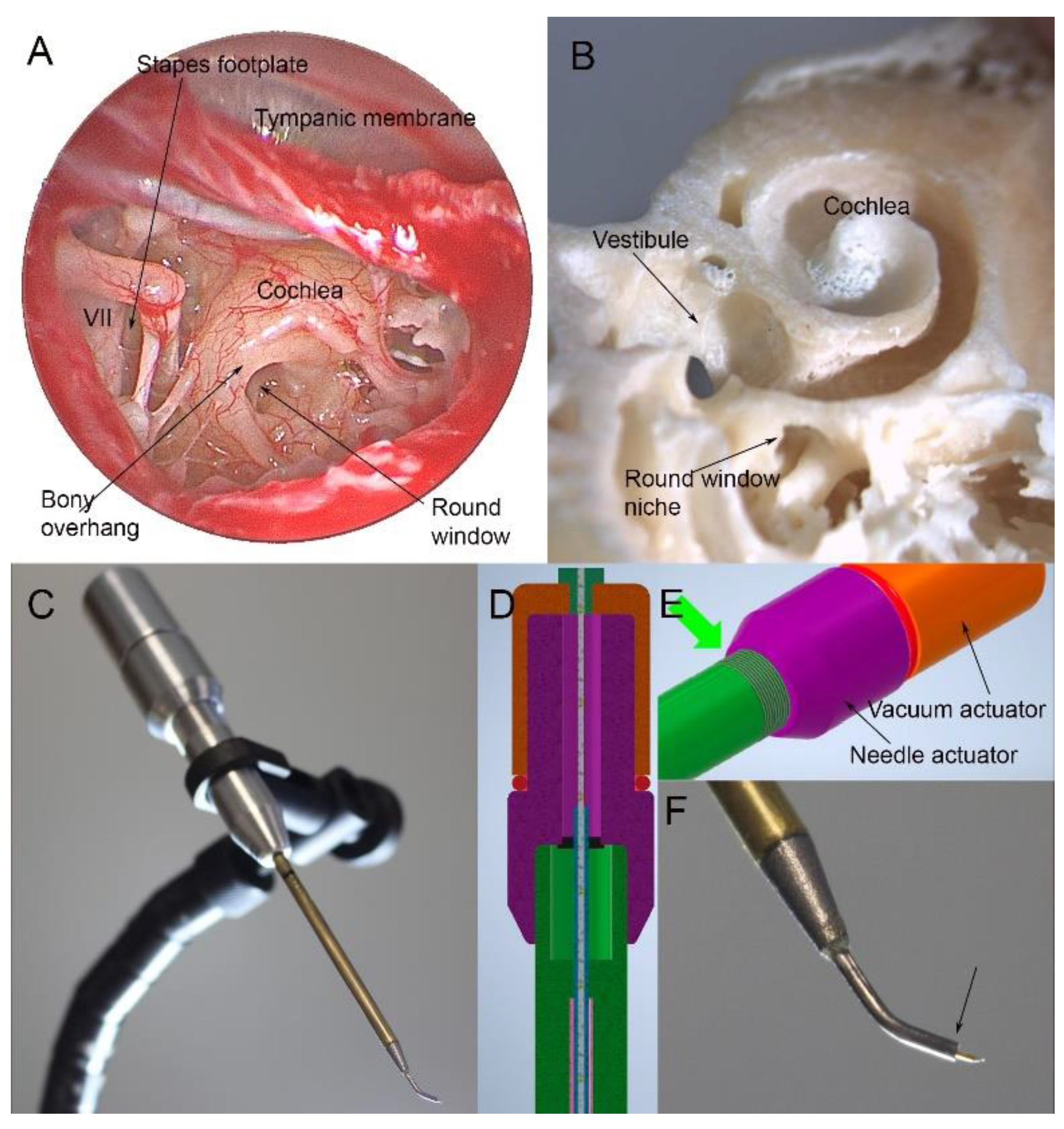This multi-sectional scientific image explores the intricacies of the human inner ear and associated surgical instruments. Section A, located in the top left, provides a circular, flesh-colored view of the inner ear featuring labels such as tympanic membrane, cochlea, bony overhang, and round window, showing the soft tissue components and vascular details. Adjacent to it in the upper right, Section B offers a cross-sectional view of the same area in stark white, depicting the bony structures, including the cochlea and vestibule, reminiscent of a skull cross-section. 

Section C, in the bottom left, displays a sophisticated surgical instrument held by a robotic arm, characterized by a black bar leading to a metallic probe, suggesting its utility in inner ear procedures aimed at alleviating pressure or performing delicate surgical tasks. 

Sections D, E, and F provide detailed close-ups and diagrams of this tool. Section D outlines the internal components, specifically the vacuum and needle actuators. Section E offers a magnified view of the tool's intricate parts, while Section F focuses on the very tip of the needle, highlighted by an arrow. The precise detailing across these sections suggests their importance in medical textbooks or resources for ear, nose, and throat (ENT) specialists.